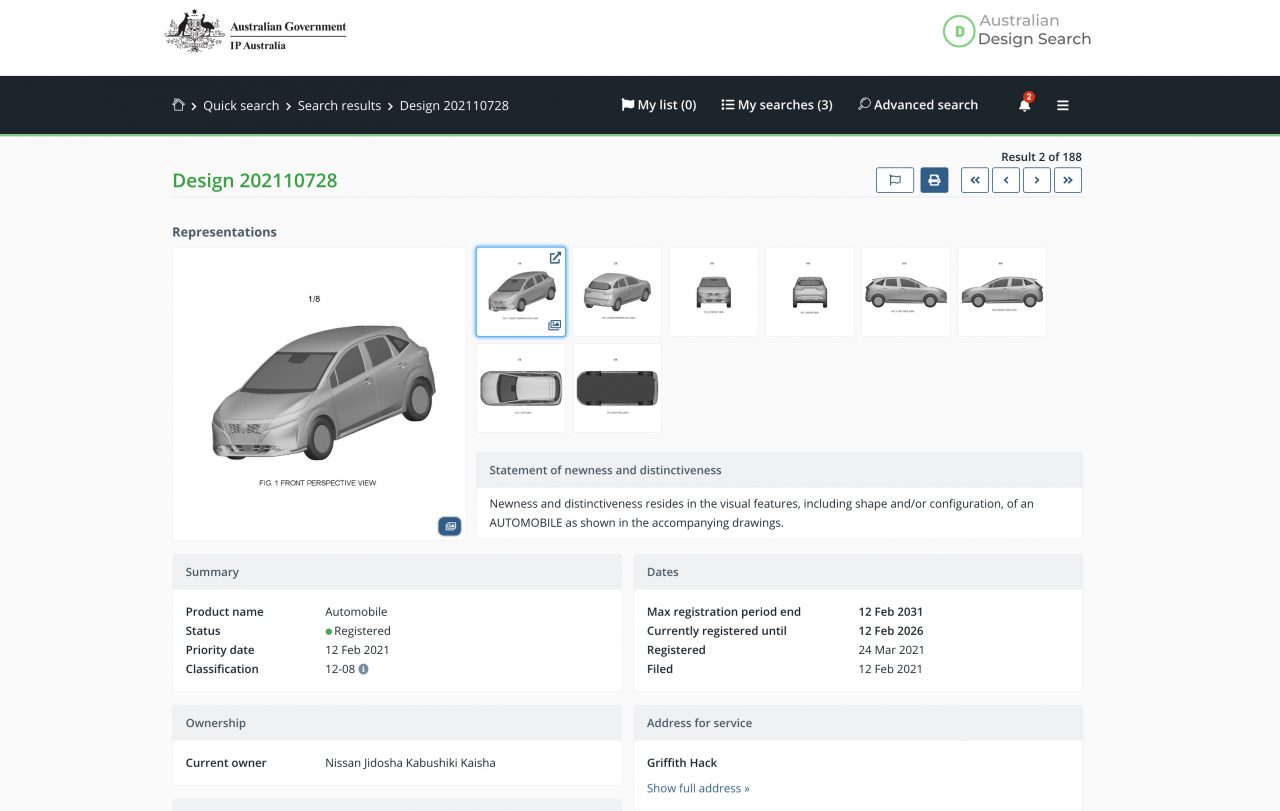This detailed color screenshot captures the interface of the Australian Design Search website, operated by the Australian Government's IP Australia. At the top left, the screen displays "Australian Government, IP Australia," while the far right reads "Australian Design Search." A black navigation banner spans the page, featuring options such as Quick Search, Search Results, Design 202-110-728, My List (0), My Searches (3), and Advanced Search. The screen indicates two notifications and highlights that the displayed result is 2 out of 188.

On the left side of the page, under the heading "Design 202-110-728, Representations," there is a computer-generated image of a dark gray car. The notation "1-8" appears above the image, with a label underneath it stating "Figure 1, Front Perspective View." To the right, numerous other images depict the car from various angles.

Beneath the images is a statement of newness and distinctiveness, which reads: "Newness and distinctiveness reside in the visual features including shape and/or configuration of an automobile as shown in the accompanying drawings."

Further down, a summary section provides detailed information:
- Product Name: Automobile
- Status: Registered
- Priority Date: 12 February 2021
- Classification: 12-08
- Ownership: Current owner Nissan Jidosha Kabushiki Kaesha
- Dates: Maximum registration period ends on 12 February 2031, currently registered until 12 February 2026
- Registration Details: Registered on 24 March 2021, filed on 12 February 2021
- Address for Service: Griffith Hack, with an option to show the full address